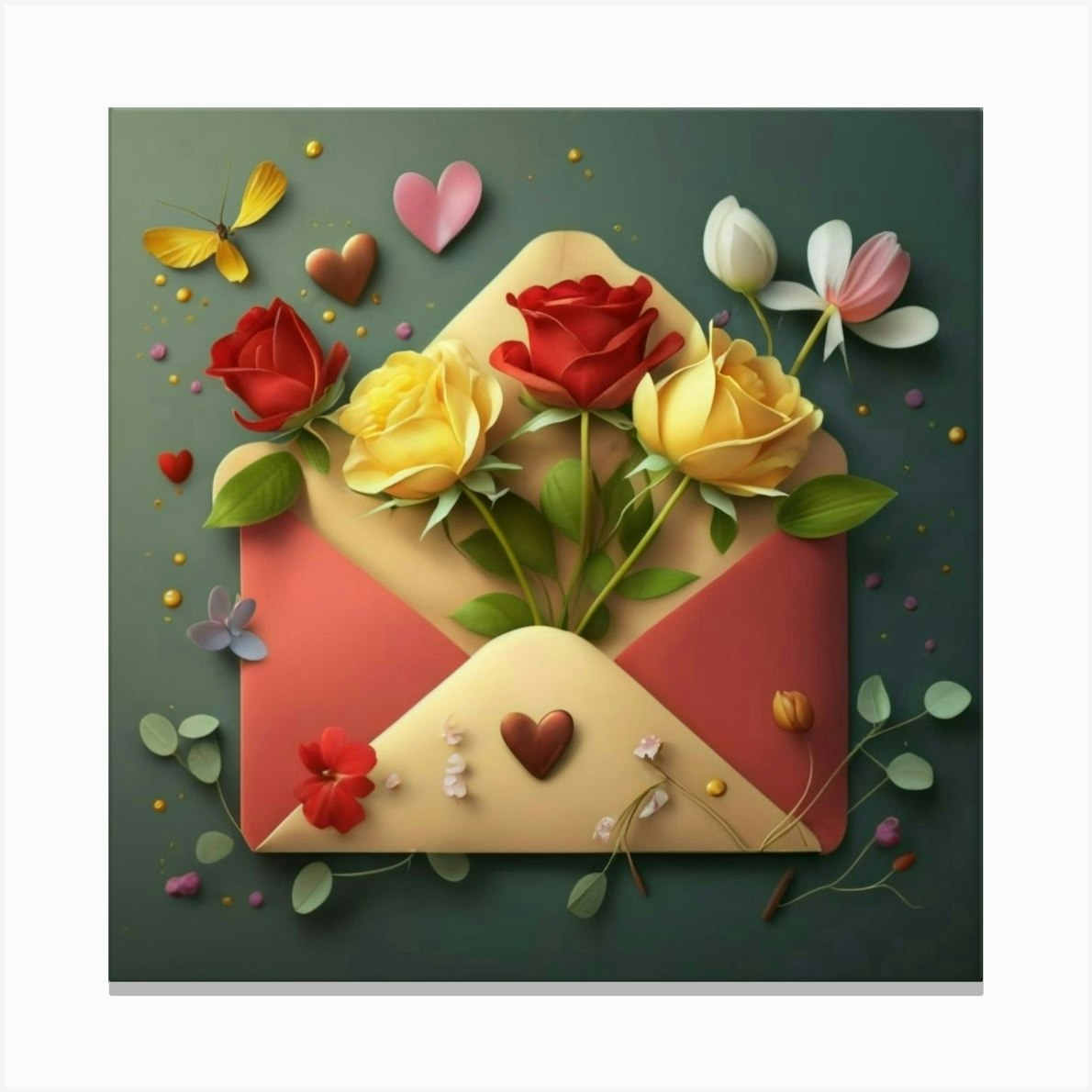The three-dimensional graphical animation showcases a vividly detailed, whimsical scene centered on an open envelope. The bottom triangle and interior of the envelope are rendered in a pale yellow, contrasting with the light red flaps on the sides. Emerging from the envelope are three main roses—two yellow roses flanking a single red rose in the center, arranged in a fan-like display. The green stems of the roses are adorned with small leaves, adding a touch of realism.

Around the envelope, the emerald green background is scattered with thin-stemmed leaves and smaller, non-blooming flowers, along with an additional red rose head positioned to the left of the envelope. The artwork is further embellished with specks of gold paint, creating circular patterns that add to the enchanting feel of the scene.

In the top left corner of the image, a butterfly, constructed from flower petals, is missing one of its bottom wings but retains two full wide wings and one pointing downward. Its antennas extend upwards at a 45-degree angle. Additionally, various colorful hearts—red, brown, and pink—are spread around the image, enhancing the visual narrative.